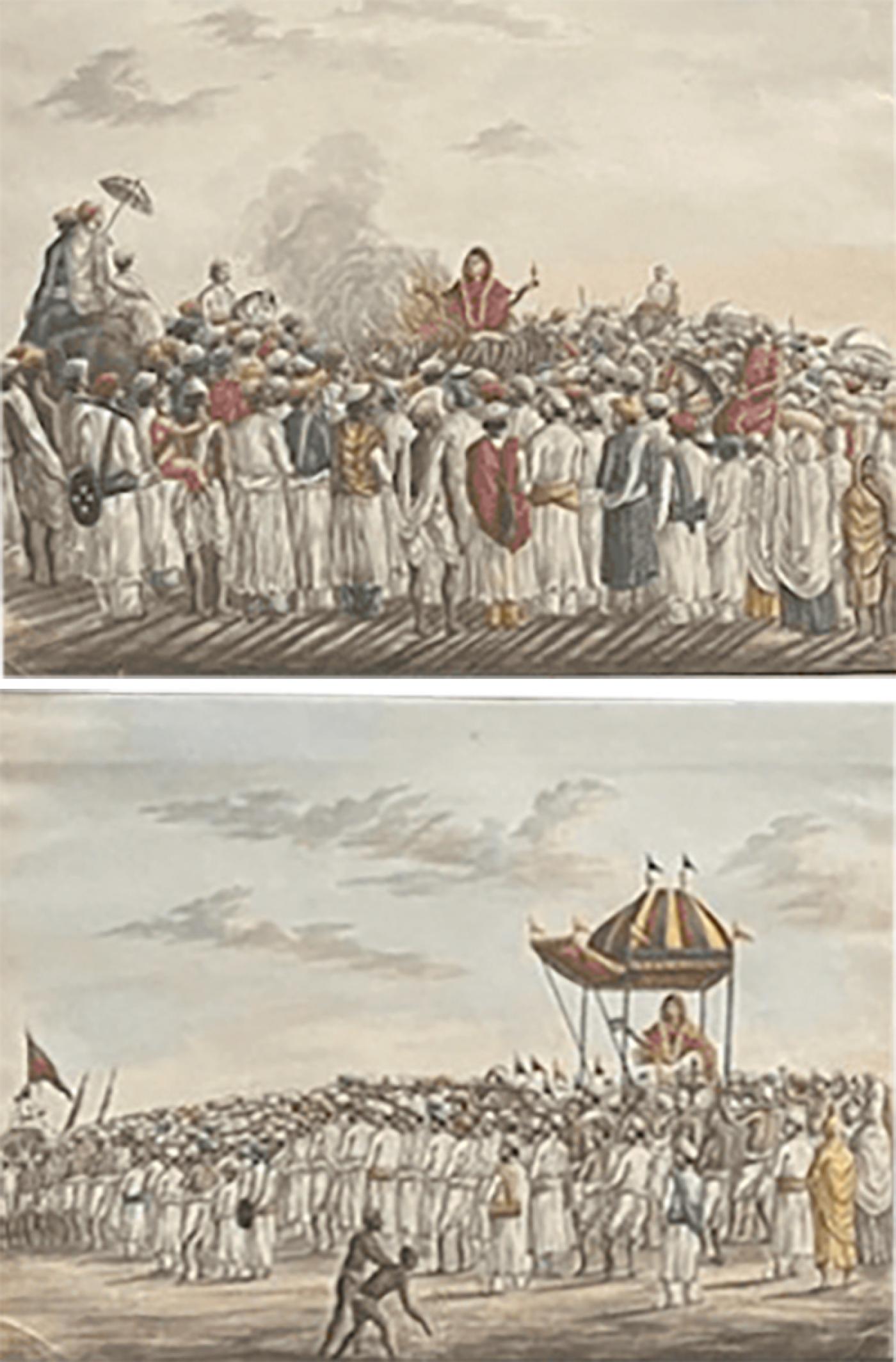The image consists of two pieces of old artwork, each depicting a religious scene with a person in a red robe with a golden cord around their neck at the center. Both paintings have foggy, smeared clouds in creamy beiges, whites, and faded reds.

In the top painting, the central figure is holding something up, surrounded by a crowd wearing traditional robes in whites, blues, reds, and a few off-yellows. The people are standing and appear to be focused on the central figure, suggesting a scene of teaching or proclamation. There is smoke rising, indicative of a fire in front of the crowd. To the left, someone is sitting with an umbrella on a rock above the crowd, accompanied by another individual.

The bottom painting shows the same central figure in the red robe, now under a small, pavilion-like structure with colorful stripes of red, blue, and yellow, adorned with small flags. The structure resembles a parasol and gives the impression of a portable throne. The crowd, mostly in white robes, is more orderly. At the far left, someone is carrying a red flag. Among the crowd, a man in yellow stands out, and noticeably, two mostly naked, dark-skinned individuals with different hairstyles are at the bottom left, contrasting with the rest of the crowd. The ground appears to be dirt with black shadows.

The overall artistic style is consistent with ancient or historical paintings, characterized by washed-out colors dominated by greys and light blues, with vibrant reds and blues accentuating key elements.